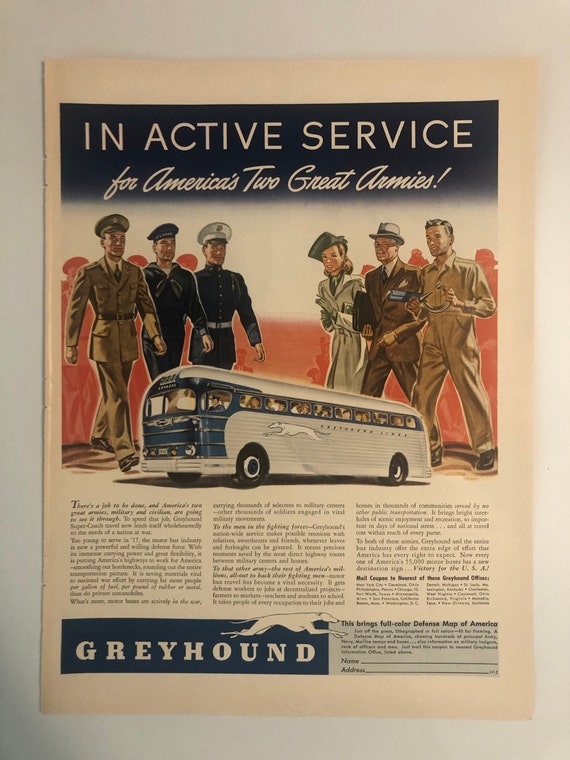This vintage poster, framed by a navy blue background, is an old-fashioned Greyhound bus advertisement. The header, in white font, reads: "In active service for America's two great armies." The central focus is a Greyhound bus prominently displaying the Greyhound logo. The scene is flanked by six figures. On the left side, we see three military personnel: an Army soldier, a Navy sailor, and what appears to be a Marine or an Air Force pilot. On the right side, stand three civilians: an actress, an older gentleman in a suit, and a mechanic. The poster underscores the unity and shared effort of both military and civilian sectors in the war effort, highlighting the role of Greyhound buses in this collective endeavor. At the bottom left corner lies another Greyhound logo solidifying the brand's presence in this patriotic-themed advertisement. The text is somewhat blurry, making it difficult to read fully, but it further emphasizes the cooperation between America's two great armies.